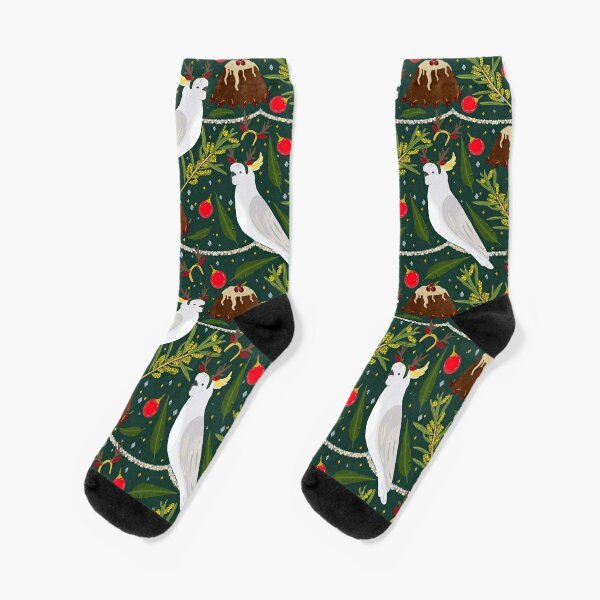This image showcases a pair of colorful holiday-themed socks, positioned side by side and centered against a light gray or off-white background. The socks are predominantly green with dark-colored toes and heels. Adorning the socks are rich, detailed Christmas motifs: a trapezoidal plum pudding with brown, white-iced topping and a cherry on top, silver tinsel strung with red Christmas balls, and various green leaves. The most striking feature is the repeated depiction of white birds, likely parakeets or doves, accented with yellow feathers on their heads and open beaks, some even donning whimsical reindeer antlers. These birds are shown roosting on rope-like lines that span across the socks. The overall composition and design evoke a festive, holiday spirit, making them ideal for a Christmas setting or product display on an e-commerce site.